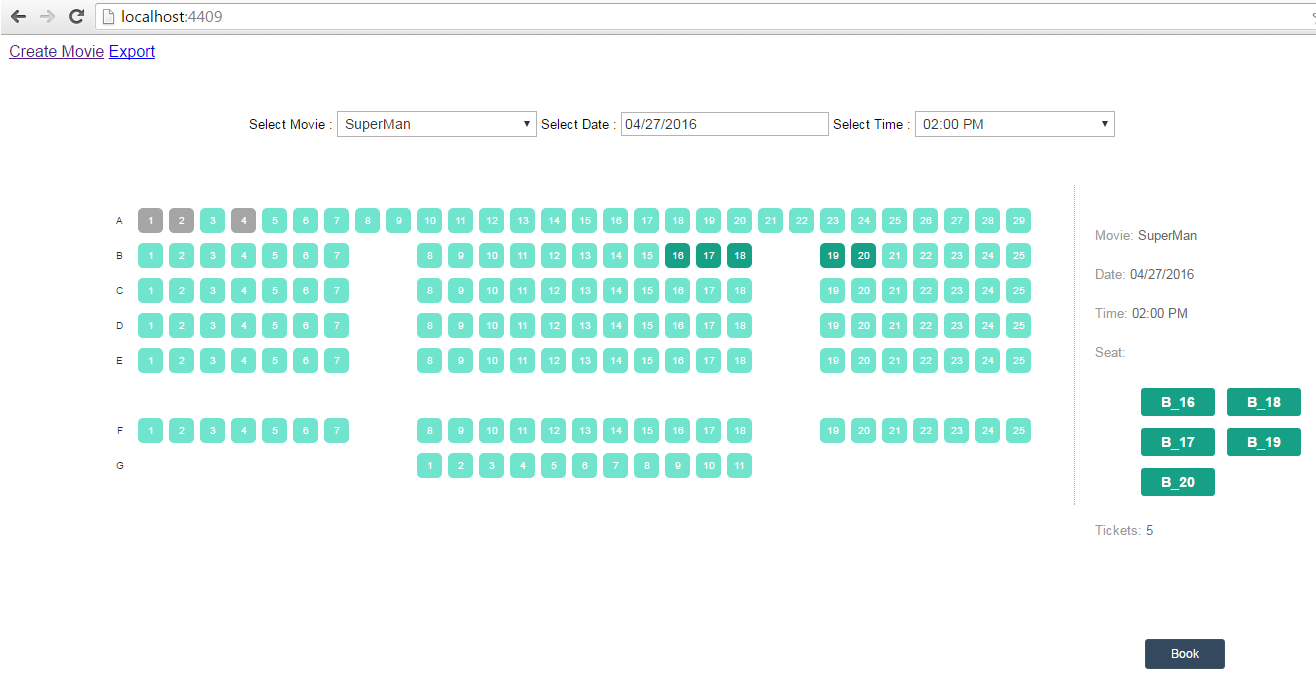Screenshot from a local web application (address bar: localhost:4409) for booking movie tickets. The interface displays options to create or export a movie, with the movie "Superman" selected. The date is set to April 27, 2016, and the time to 2 p.m. In the center of the interface, there is a detailed seating chart with rows labeled from A to G. Seats A1, A2, and A4 in the first row are selected, as well as seats B16, B17, B18, B19, and B20 in the second row. The booking summary shows the movie "Superman," with the specified date, time, and selected seats in row B (B16-B20), indicating a total of 5 tickets. At the bottom of the interface, there is a black button with the word "Book" in white letters. The image contains no people, photographs, plants, trees, vehicles, or any other elements outside the booking interface.